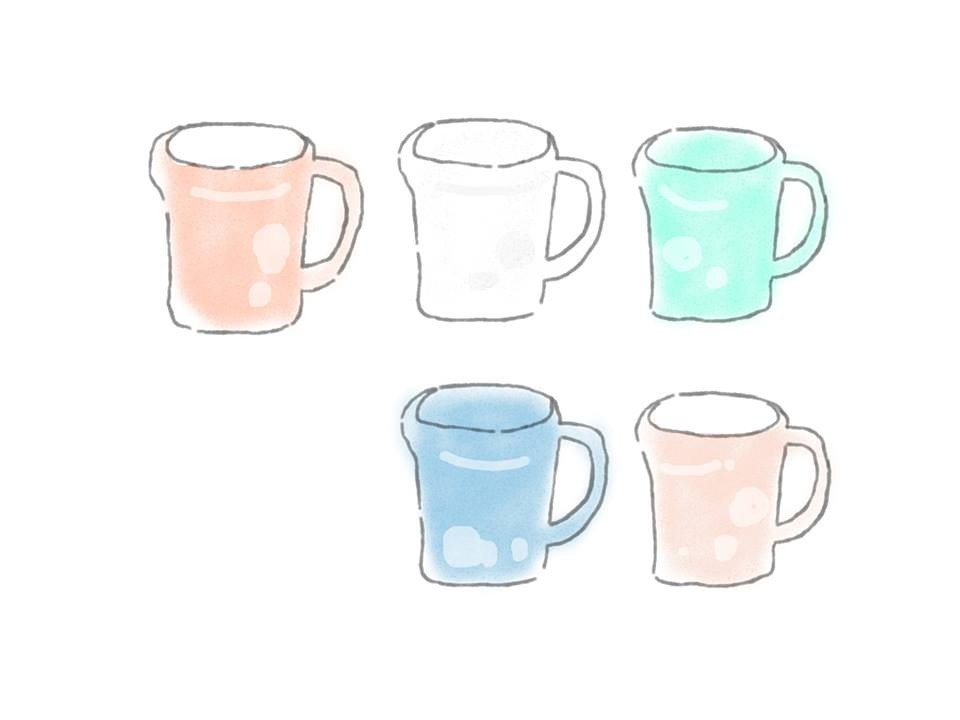This image is a colored drawing of five coffee mugs, arranged in two rows against a plain white background. The bottom row features a blue mug on the left and a soft pink mug on the right. The blue mug has a handle that’s also blue, while the pink mug has a white top. The top row consists of a very light blue-green mug on the right, a white mug in the middle, and a light red or dark pink mug on the left. Each mug is outlined with black lines and is decorated with faded circular shapes suggesting a glare. Although most mugs are white inside, the blue mug on the bottom row and the light blue-green mug on the top row are shaded completely. The drawing uses a simple yet detailed style, giving a watercolor-like appearance to the colors. The mugs appear as if they might contain beverages, enhancing their lifelike depiction from a frontal view.